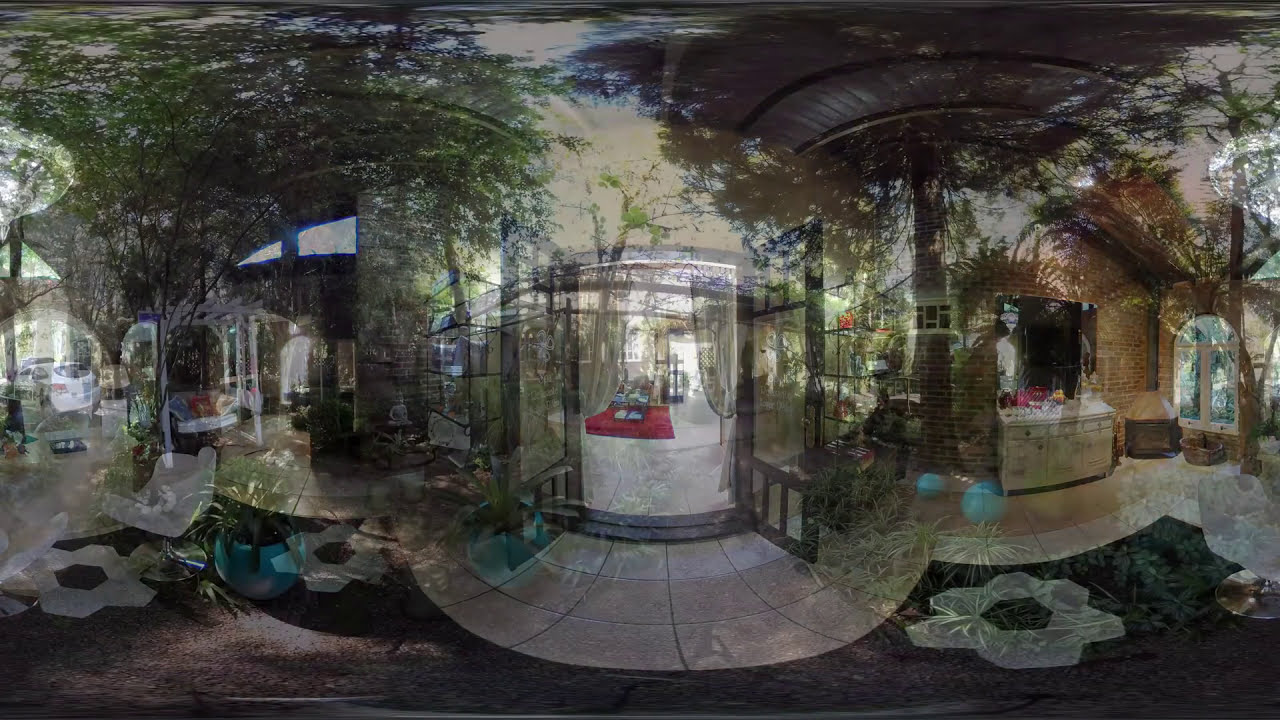The photograph captures an intricately designed outdoor garden or patio area, located in what seems to be an urban or city street setting. Dominating the center of the image are two wide, open glass doors framed in black, giving a glimpse into an interior section. The doors themselves are rectangular with black panels, and within this frame, a red square and other faint, indistinguishable images can be seen. Overhead, tree canopies extend from both the left and right sides, contributing to the lush greenery that pervades the scene.

On the left side, a tree with abundant leaves stretches out, while on the right, a larger tree is accompanied by several smaller ones. The foreground features a distinctive scalloped walkway, composed of light gray cement tiles, with the central scallop extending towards the viewer and additional scallops radiating outward to the left and right. This area is dotted with white, flower-like patterns or designs, possibly made of film or nylon, blending seamlessly with the walkway.

To the right of the walkway, a tree is visible along with what appears to be a seating area, and further back, there seems to be another patio or lobby area with a desk or table, although the objects on it are unclear. On the left side of the image, an indistinct street runs parallel to the scene, adding to the urban atmosphere. Overall, the photograph is a harmonious blend of natural elements and urban design, enriched with diverse patterns and textures.